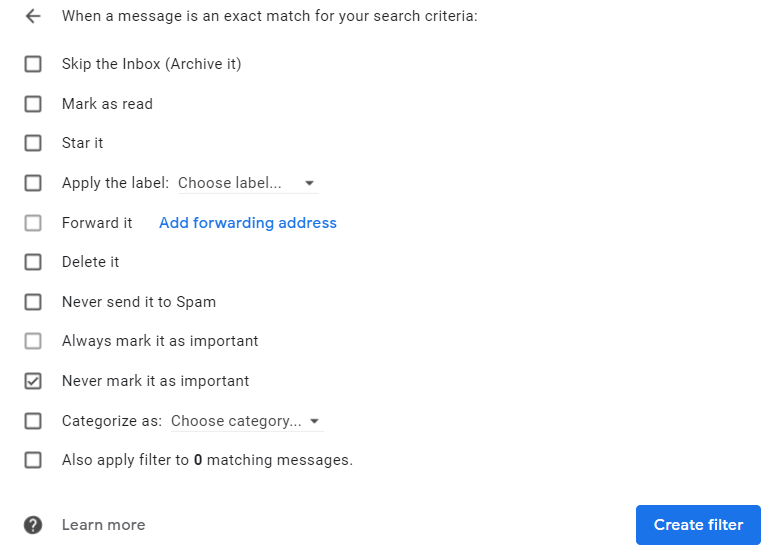This image is a screenshot of a dropdown menu from a computer interface with an all-white background. At the very top, there's a left-pointing arrow followed by the text, "When a message is an exact match for your search criteria:". Below this heading, a series of options is presented with checkboxes next to each.

1. **Skip the Inbox (Archive it)**
2. **Mark as Read**
3. **Star it**
4. **Apply the label: [Choose label]** (contains a dropdown box)
5. **Forward it** (with "Add forwarding address" in blue text next to it)
6. **Delete it**
7. **Never send it to Spam**
8. **Always mark it as important**
9. **Never mark it as important** (this option has a checkmark next to it)
10. **Categorize as: [Choose category]**

Beneath these options, there's text stating, "Also apply filter to zero matching messages". At the very bottom of the dropdown, there is a black circle with a question mark inside it and the text "Learn more" next to it.

Notably, the "Never mark it as important" option is the only one checked. Additionally, the "Forward it" and "Always mark it as important" options appear slightly lighter in color, indicating they are possibly disabled or inactive.